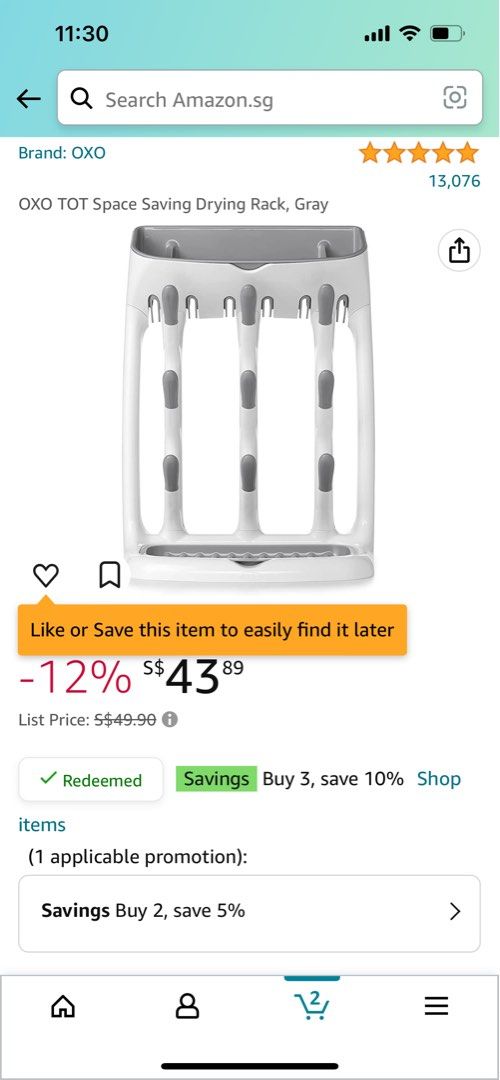**Detailed Caption:**

This is a detailed screenshot of an Amazon shopping page, presumably from a foreign country, given the currency symbol used. The image is in portrait orientation, resembling a typical cell phone screen with a significantly taller than wide proportion. 

- **Top Bar:** At the very top, there is a lightish blue and green gradient border that fades into a teal color. Within this rectangular box, the time is displayed as "11:30" in black. To the right of the time, there are three icons: 
  - A network connection icon which is fully filled,
  - A Wi-Fi icon also shown as fully connected,
  - A horizontal battery icon displaying a black meter more than half full.
  
- **Navigation and Search:** Below this top bar, a black left-pointing arrow is visible, likely for navigation purposes. Adjacent to the arrow, there is a white rectangular search box with the placeholder text "search Amazon.sg" in grey font, indicating this might be the Singapore version of Amazon.

- **Product Information:** The section below the search box features product details against a white background:
  - The product brand is displayed in blue font as "OXO," followed by five gold stars with "13,076 ratings" written underneath.
  - The product description in grey font reads "OXO Tot Space Saving Drying Rack, Grey," accompanied by a clear image of the item. 
  - Beneath the image, there are two interactive buttons: a "like" button and a "bookmark" button.

- **Pricing Details:** An orange rectangular border encloses the price information:
  - It states a discount of "Minus 12%" for the product, bringing the price down to "S$43.89," indicating that the currency is Singapore dollars.
  
- **Additional Savings Information:** Below the price, a white box with green font and a green check mark displays the message "redeemed," showing additional savings of 3.10%.

- **Shopping Cart:** At the bottom of the screenshot, an icon of a shopping cart is visible with a notation indicating there are two items currently in the cart.